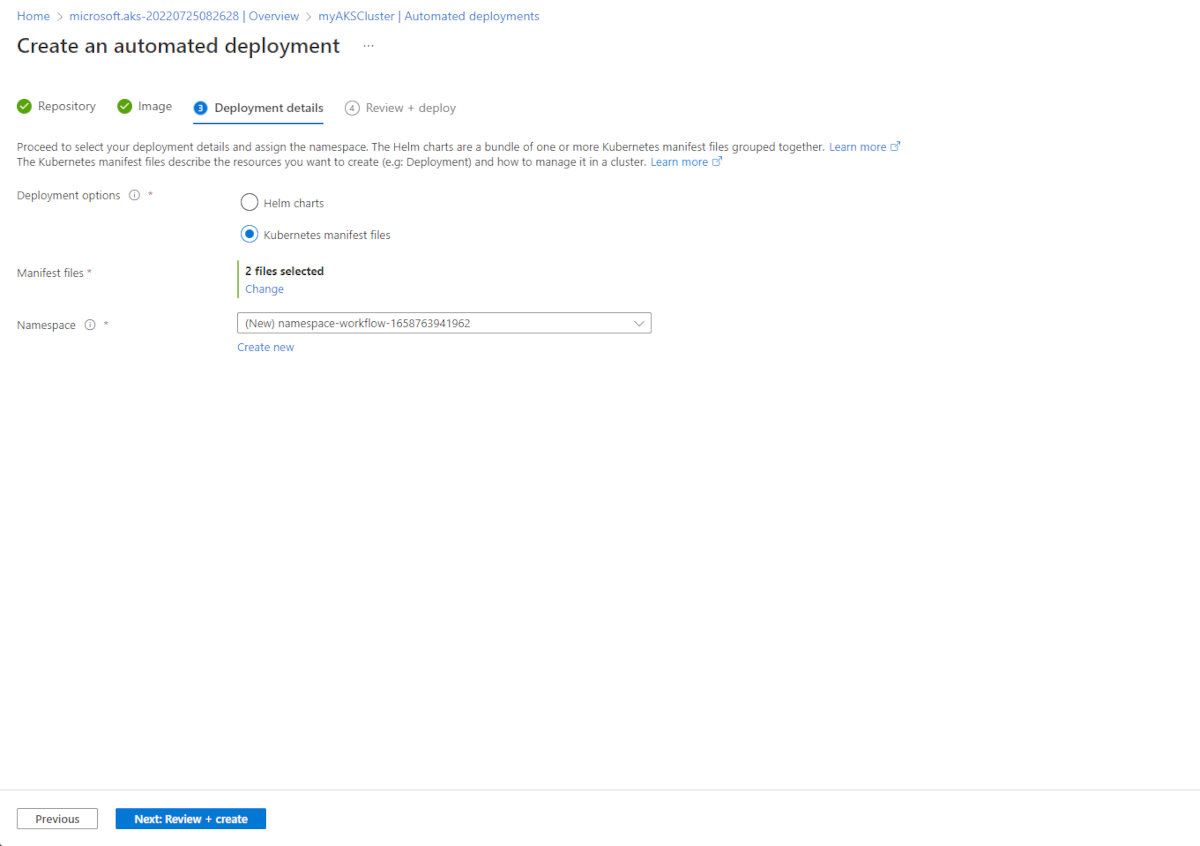**Detailed Caption:**

The detailed image depicts a user interface from Microsoft's Azure Kubernetes Service (AKS). In the top left corner, the navigation path is visible, starting with "Home," followed by "Microsoft.AKS," a series of numbers, and continuing through to "Overview," "My AKS Cluster," and finally landing on "Automated Deployments."

The main header reads "Create an Automated Deployment" in bold text. Below it, there are four tab headers indicating steps in the deployment process. The first two steps, "Repository" and "Image," are marked complete with green check marks. The third tab, "Deployment Details," is highlighted with a blue circle containing the number three and is underlined in blue. The fourth tab, marked with a number four in an open circle, is still pending.

The central section of the page discusses "Deployment Details." Instructions guide the user to select deployment details and assign the namespace. There is a brief explanation about Helm Charts as bundles of one or more Kubernetes manifest files, with a blue "Learn more" link offering additional information. It further describes that these manifest files are used to describe desired resources and their management within a Kubernetes cluster, also with a "Learn more" link in blue.

On the left side of the screen, options include "Deployment Options," "Manifest Files," and "Namespace." On the right, there is a toggle button allowing the choice between "Helm Charts" and "Kubernetes Manifest Files," with the latter selected. Underneath, bold text indicates "Two Files Selected," with an option to change this selection available.

Further down, there is a "New Namespace Workflow" drop-down menu with the option to "Create New" highlighted in blue. At the bottom of the interface are two navigation buttons: a "Previous" button, and in blue, a "Next: Review and Create" button.

Overall, the image provides a clear step-by-step guide through the automated deployment setup in AKS, highlighting the current stage and actions required for successful configuration.